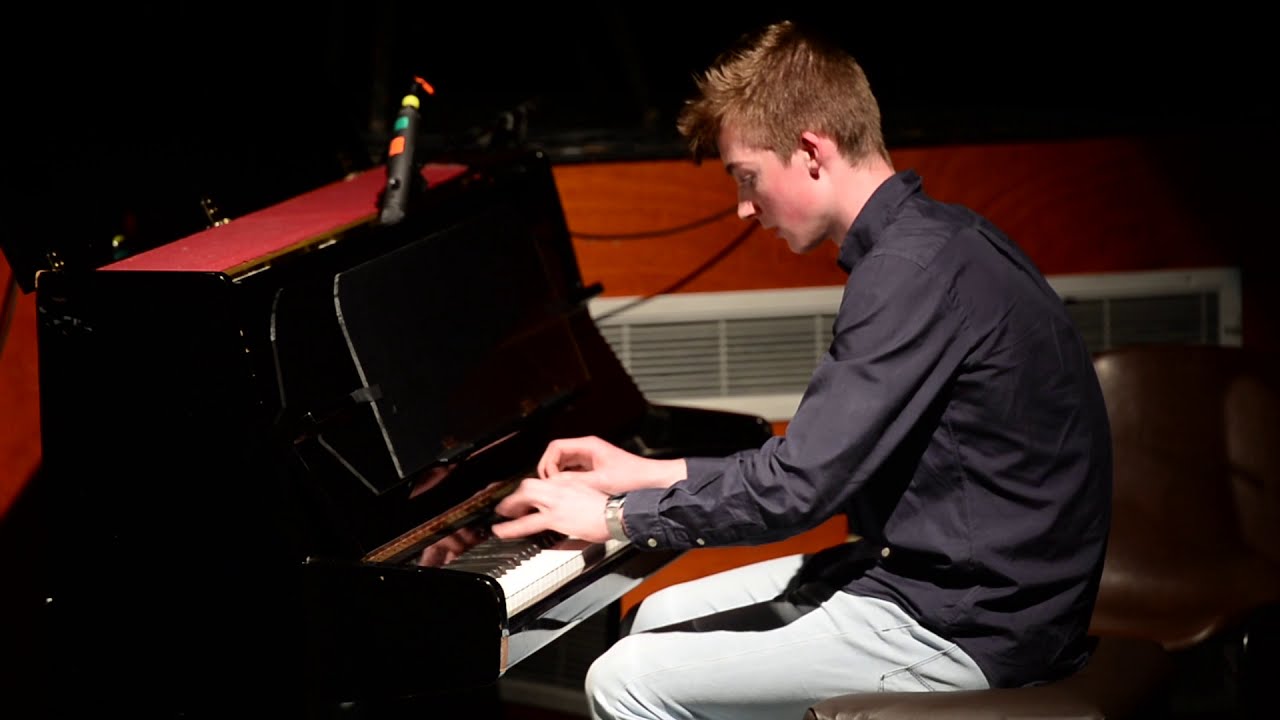The image depicts a young boy, likely in his early teens, intensely focused on playing a black, glossy upright piano positioned somewhat diagonally on the left side of the frame. He is seated on a brown bench facing left, with both hands hovering over the keyboard, fingers poised over the black keys. The boy is dressed in gray dress pants and a dark bluish-gray long-sleeve button-up polo shirt, his short brownish hair slightly bent towards the keys. The piano, which has a velvet covering and no sheet music, features a black contraption on top adorned with orange, green, yellow, and red elements. The backdrop of the scene is a red wall with a white, elongated horizontal radiator. Additionally, there is a hint of a performance setting, suggested by directed lighting and a stage platform behind the boy.